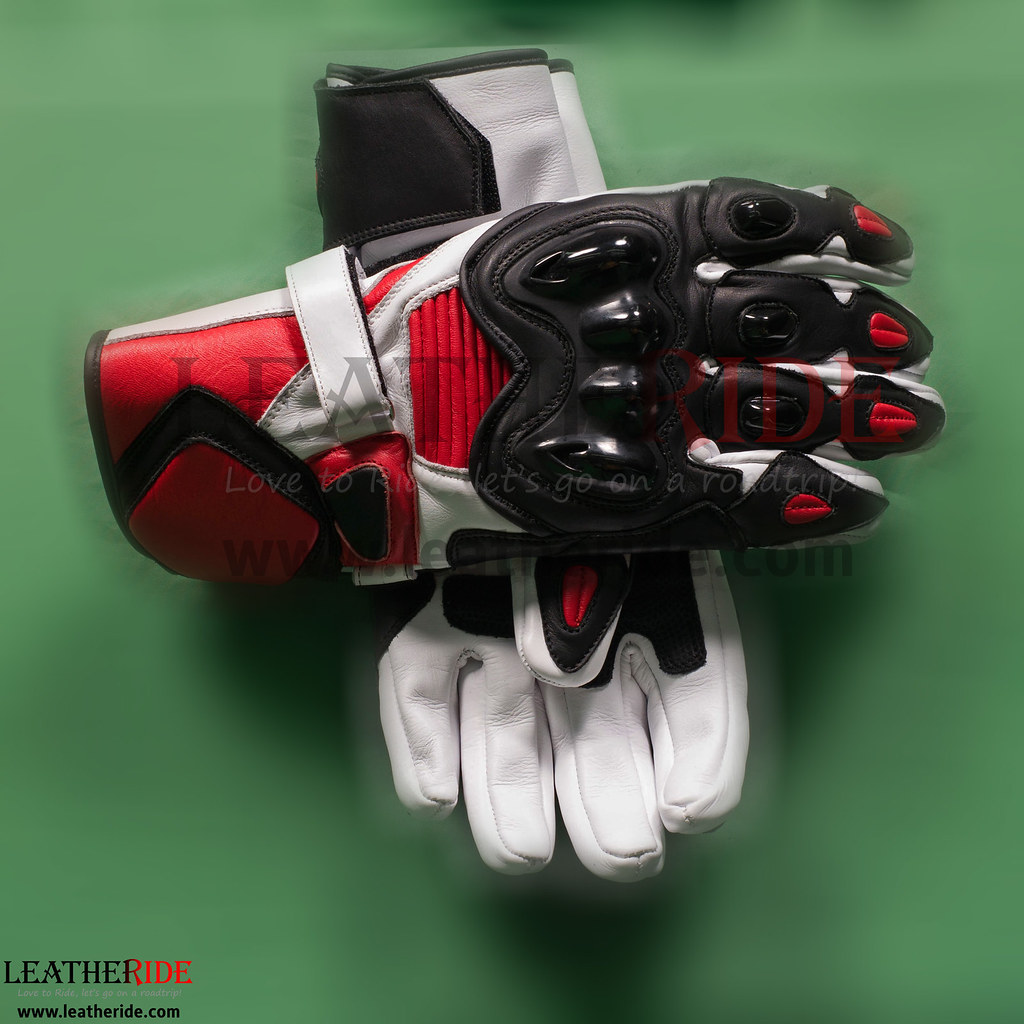This image showcases an advertisement set against an olive green backdrop. Dominating the center are two black, red, and white leather gloves positioned with one vertical and the other horizontal. These gloves feature intricate design details, including raised plastic bumps on the knuckles and fingertips, ensuring enhanced protection and comfort. The gloves also have distinctive white straps around the wrist areas, providing a secure fit with a potential Velcro closure. The central top portion of the gloves is red while the underside is predominantly white with black accents.

At the bottom left of the image, "Leather Ride" is prominently displayed, with "leather" in black and “ride” partially in black and red. Beneath this text is smaller gray writing, too small to decipher, followed by "leatherride.com" in black. Overlaying the center of the image is a watermark for "leatherride.com" accompanied by the slogan "Love to ride. Let's go on a road trip" in white text.